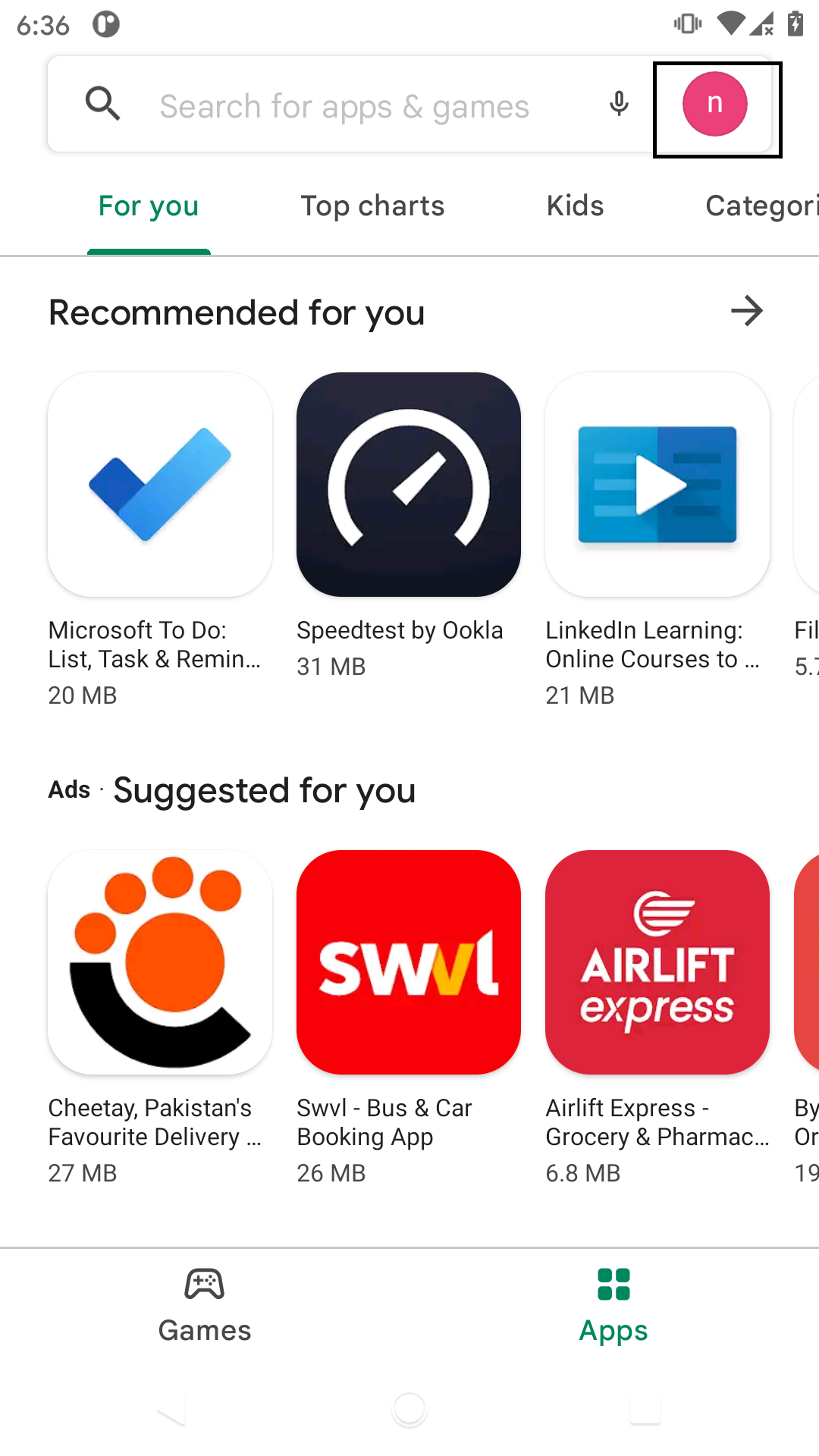A detailed screen capture from what appears to be an app store interface, presumably viewed on a tablet due to the wide screen display, though it could also be on a phone. The top of the screen features a search bar labeled "Search for apps and games." The device clock shows 6:36, and the battery is fully charged.

Beneath the search bar, several navigation tabs are visible: "For you," "Top charts," "Kids," and "Categories." Below these tabs, a "Recommended for you" section features a selection of apps: "Microsoft To Do List, Task and Reminders," "Speedtest by Ookla," and "LinkedIn Learning, Online Courses." Each listing includes the size of the app, indicating that they are relatively small.

Further down, an "Ads suggested for you" section is presented, showcasing apps such as "Cheetah, Pakistan's Favorite Delivery," "SWVL, Bus and Car Booking App," and "Airlift Express, Grocery and Pharmacy." At the bottom of the screen are two more tabs labeled "Games" and "Apps," offering additional categories for navigation.